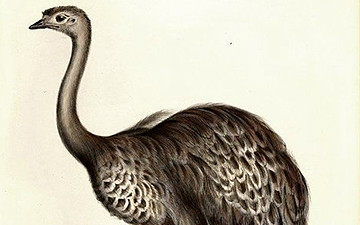This is a highly detailed hand-drawn portrait of a bird resembling either an ostrich or a turkey. The bird is characterized by its long neck, relatively small head, and short beak, with one visible eye emphasizing its expressive gaze. The drawing showcases intricate details in the feathers, which are depicted in shades of brown with white highlights, giving a sense of depth and texture. The bird appears to be mid-sized, larger than a sparrow but not overwhelmingly huge, and is presented in a side view facing towards the left. The background of the artwork is a plain cream or tan color, likely meant to emphasize the bird, with no additional elements such as text, dates, or people. The medium used for this drawing could be lead or graphite on a possibly yellowish parchment-type paper. The overall dimensions of the image are quite small, approximately two by two inches, suggesting limited but deeply focused information within the frame. The bird's feathers hang down thickly, contributing to the detailed and shaded depiction of its plumage, and the upright posture, although legless in this view, adds to the striking composition centered solely on the bird.